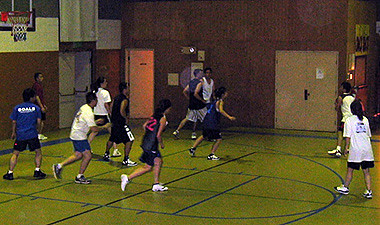This small, grainy, and rectangular image captures a vibrant scene of a co-ed basketball game played by teenagers inside a gymnasium. The court has a striking lime green hue with blue lines marking the play areas, giving it a polished and well-maintained appearance despite the image's lack of vividness. At the top left corner, a basketball backboard with a blue border and white lines is visible. The photograph shows five players on the left side in motion, seemingly running towards the right, where other players have their backs turned. The athletes are wearing casual athletic clothes, with one team donning blue shirts and the other in white. The gym features several doors: an open door on the left background, a double door on a brick wall to the right, and two closed double doors on the back wall to the left. The game is energetic, with most players airborne or in dynamic poses, though the basketball itself is not visible. The colors of the photo suggest it may be older, as the gym floor has a distinctive greenish cast, adding to the image's nostalgic feel.